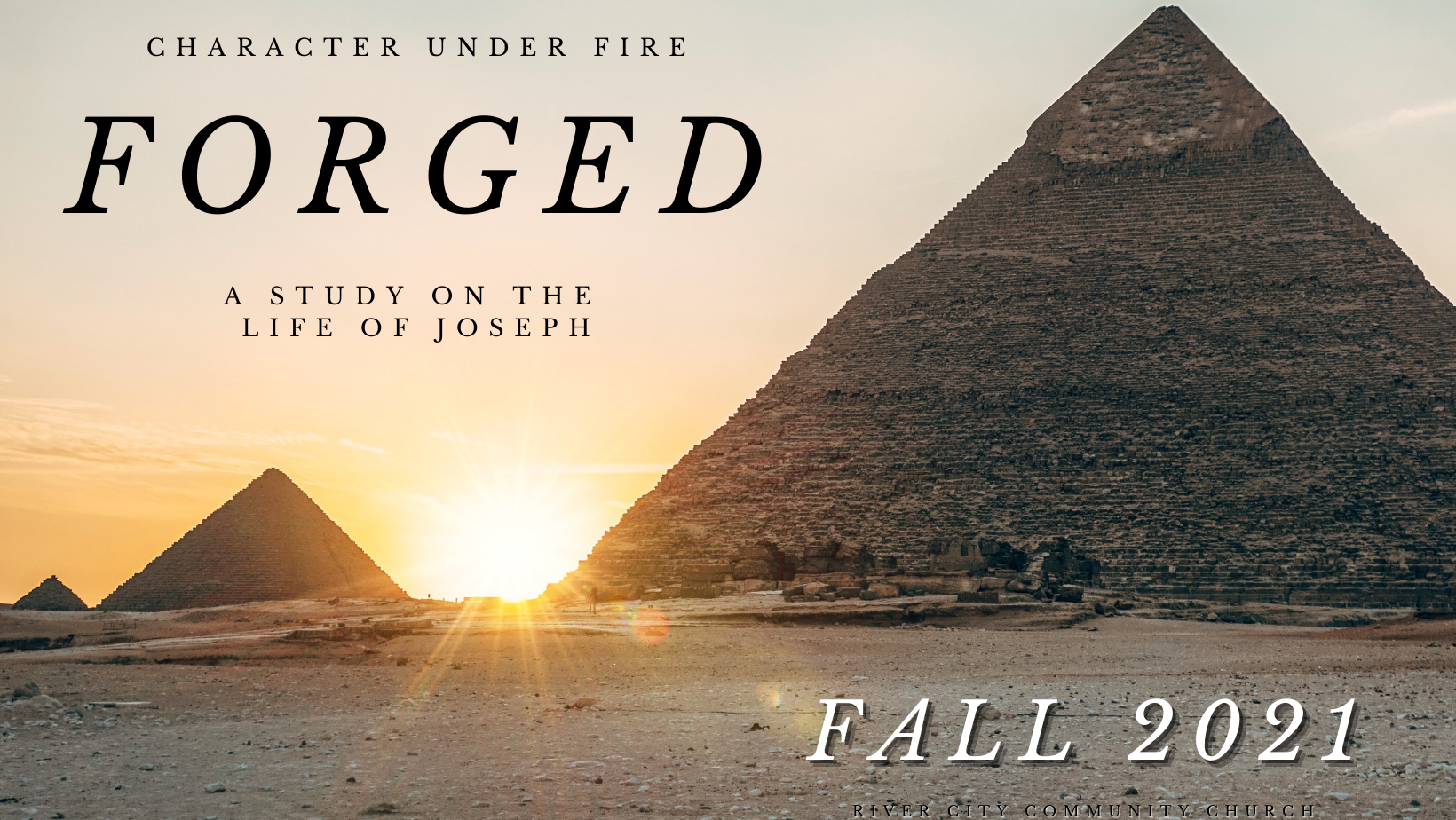The image appears to be an advertisement for a study on the life of Joseph titled "Character Under Fire: Forged." The cover showcases a stony, sandy desert landscape featuring three pyramids arranged in a line. The largest pyramid stands on the right, with a smaller pyramid in the center and another in the background. Between the largest and the central pyramid, the sun is either rising or setting, casting its rays across the scene and creating a picturesque view. The sky above is light gray with a few clouds, tinged yellow by the sunlight. The overall effect gives a historical and ancient feel to the image. The words “Character Under Fire: Forged, A Study on the Life of Joseph,” along with the date “Fall 2021,” are prominently displayed, suggesting an enriching exploration of historical insights through Joseph’s story.